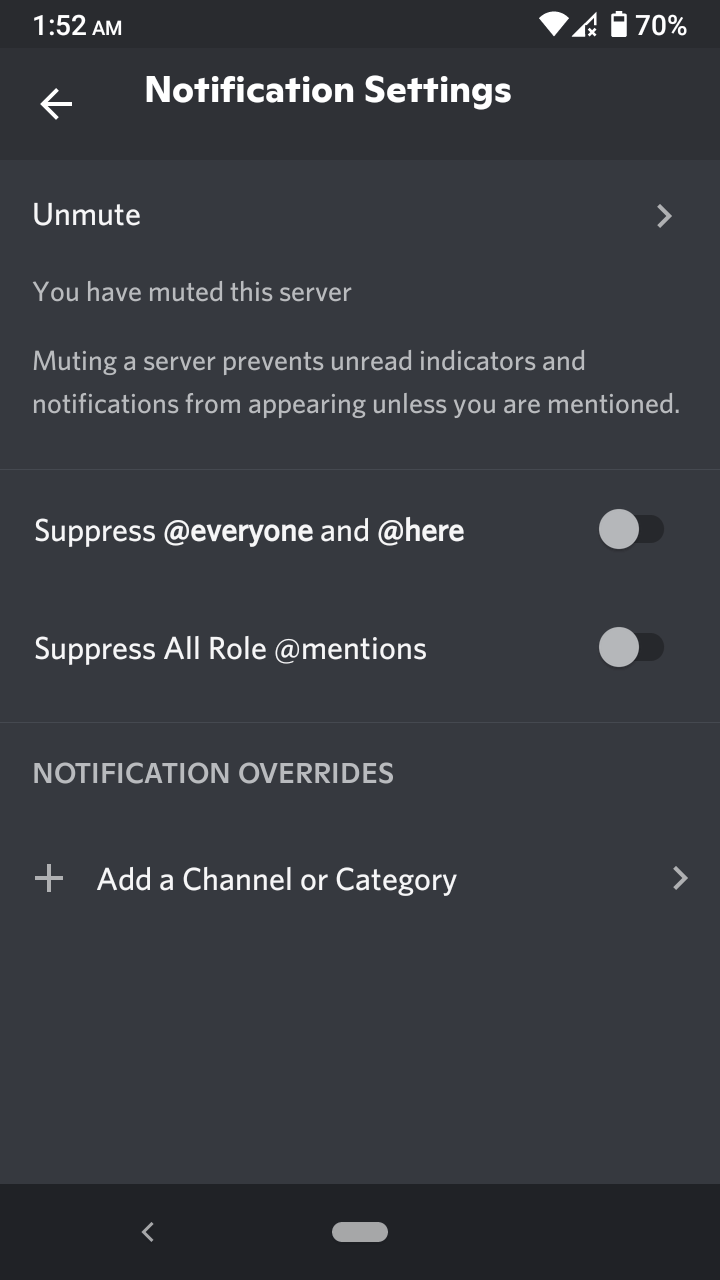The image displays the settings section of a mobile application on a phone, featuring a dark theme with a black and dark grey background and white text. The top of the screen provides various status indicators for the device: the time is shown as 1:52 AM in the top left corner, while the right corner displays Wi-Fi, network connection symbols, and a battery icon indicating 70% charge.

The main title of the screen reads "Notification Settings." The first option listed is "Unmute," accompanied by a right-facing arrow for accessing more options. Below that, a message informs the user, "You have muted this server. Muting a server prevents unread indicators and notifications from appearing unless you are mentioned." 

Further down, the settings include toggles for two particular features. "Suppress @everyone and @here" is followed by an on-off switch currently set to off. Similarly, "Suppress all role @mentions" has an off position as well. At the bottom of the screen, the section titled "Notification Overrides" appears, featuring a plus symbol next to "Add a channel or category," with a right-facing arrow for additional options.